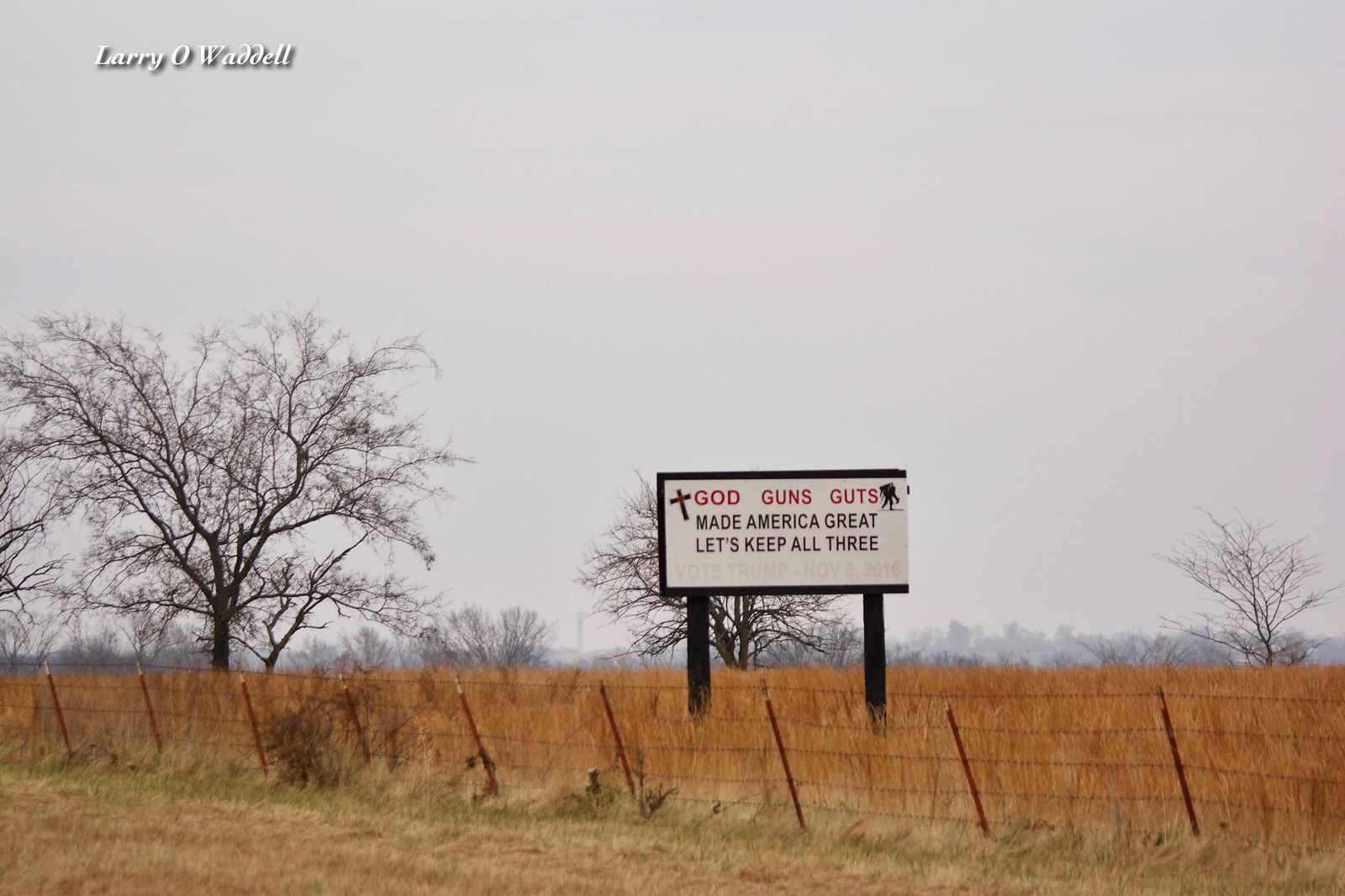In this roadside scene, a vast field of tall, brown grass stretches out, bordered by a wire fence with striking red poles. Two prominent, bare trees stand amidst the field, their branches stark against the sky, while other leafless trees form a sparse backdrop. Scattered around the field are several black poles and a distinct black outline. At the forefront, a white sign captures attention with its prominent red and black lettering. The sign features a cross and reads, "God, Guns, and Guts" in bold red letters. Below, in smaller black text, it proclaims, "Made America Great, Let's Keep All Free." A small, unobtrusive black hole punctuates the lower part of the sign, adding a curious detail to this striking and evocative roadside display.